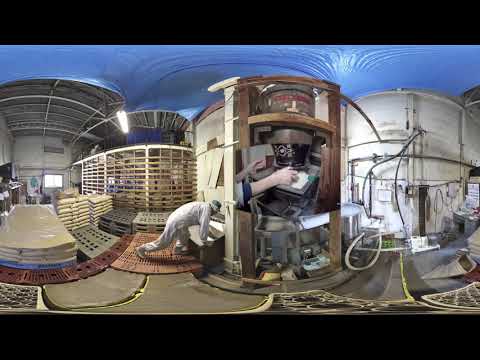The image is a heavily distorted panoramic photograph or video frame of an industrial workspace, likely a textile plant or factory with a fisheye lens effect. Bound by thin black bars at the top and bottom, the scene curves in a surreal manner. The central focus is a man in an all-white suit, possibly a hazmat suit or industrial coverall, and a gray hat. He is leaning towards a piece of industrial equipment that appears to be a large wooden press or stamping machine with a significant black barrel in the center, seemingly engaged in moving or manipulating some material. The floor, a peculiar brown with odd curves, adds to the distorted effect. The left side reveals a warehouse with light greenish-gray walls, several stories high, supported by metallic beams. There are stacked crates and gray bags on shipping pallets, and a wooden fence-like structure. The far right of the image shows a white wall with numerous hoses, wires, and electrical conduit, creating a chaotic backdrop. Above, a foamy blue ceiling looms overhead, potentially indicating a loading dock area. To complete the scene, there's a window emitting light, adding to the industrial ambiance.